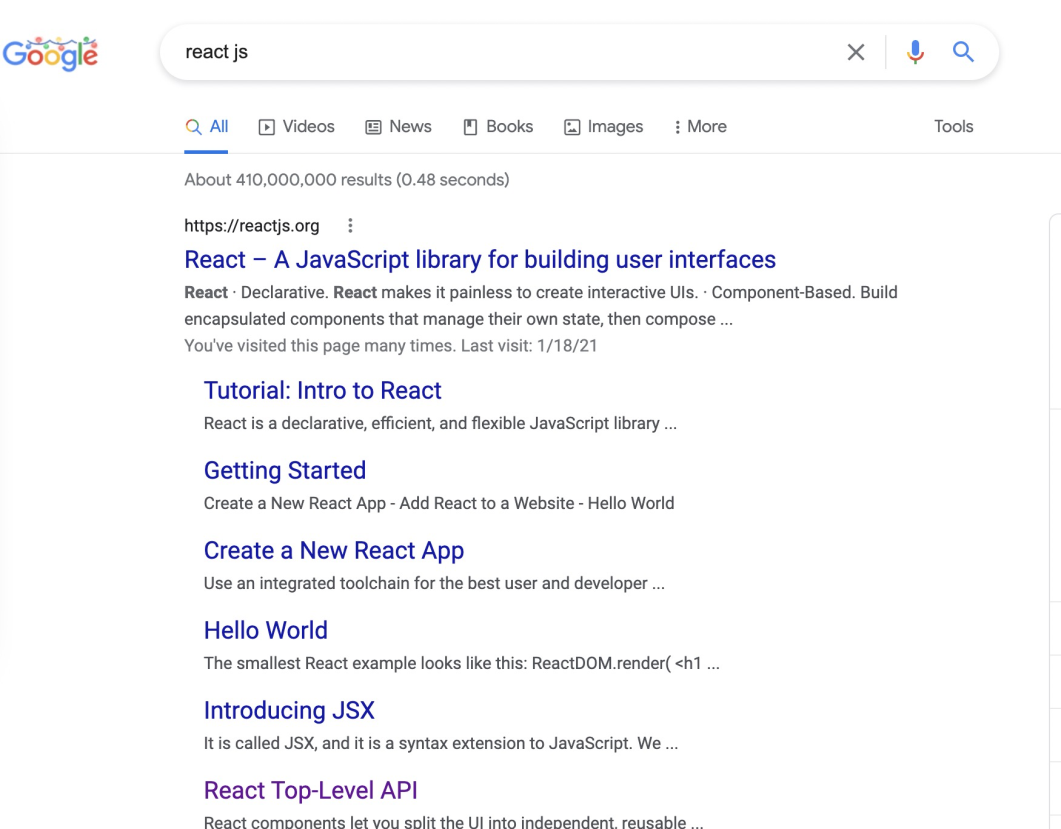A Google search results page for "React JS" is displayed. In the top left corner, the Google logo is adorned with festive Christmas decorations, indicating the holiday season. The search bar at the center of the header shows the keyword "React JS" with a microphone icon on the right for voice search and a magnifying glass icon for initiating the search.

Below the search bar is the navigation menu starting with "All," followed by "Videos," "News," "Books," "Images," and "More." The search results indicate about 410 million entries found in 0.48 seconds.

The first search result links to "reactjs.org," the official documentation for React, which is described as a JavaScript library for building user interfaces. Snippets from the site highlight React’s declarative approach, making UI creation painless and component-based architecture, enabling encapsulated components that manage their own state. A note mentions the user has visited this page many times, with the last visit dated January 18, 2021.

Additional information from the same link offers a tutorial introduction to React, emphasizing its efficient and flexible nature. It suggests starting by creating a new React app and integrating React into an existing website, mentioning "Hello World" as the simplest example. The tutorial also covers using the integrated toolchain for an optimal user and developer experience and introduces JSX, a syntax extension for JavaScript employed by React.

In summary, the image captures a typical Google search results page with detailed insights and examples from the React.js official site, providing a starting point for both new and experienced developers looking to utilize this powerful JavaScript library.